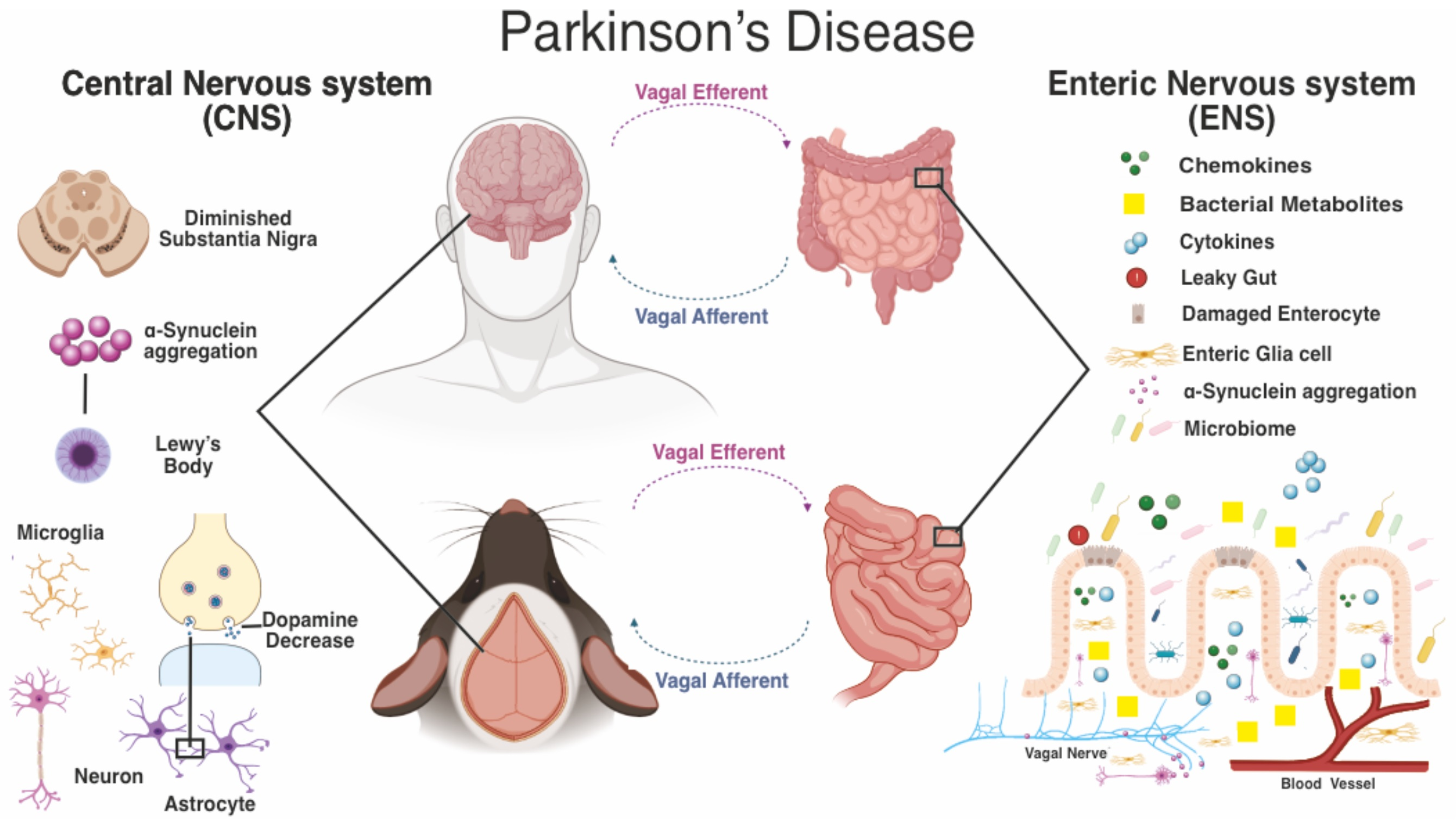This digital infographic on a plain white background explores Parkinson's disease through a series of detailed, color-illustrated diagrams and textual labels. At the top center, the title reads "Parkinson's disease" in black text. On the left side, the subtitle "Central Nervous System (CNS)" is displayed, and on the right, "Enteric Nervous System (ENS)" is indicated. 

Beneath the main title, the top-left section features an outlined human figure from the shoulders up, with a detailed brain visible inside the head. A black line connects this brain to an adjacent diagram of a mouse's head, shown from a top-down view, highlighting its brain. Toward the right of the human head illustration, there's a detailed drawing of the gastrointestinal (GI) system, showcasing both large and small intestines. A black box highlights a part of the small intestines, from which another line leads to a blown-up section of what appears to be pink small intestine tissue. This tissue section is annotated with terms like "vagal efferent" and "vagal afferent" multiple times.

Further to the left under the CNS subtitle, additional diagrams illustrate specific elements like "diminished substantia nigra," "α-synuclein aggregation," and "Lewy bodies." On the right, under the ENS subtitle, you find a legend and icons with accompanying titles, helping to clarify the details in the images, such as parts of the brain and other organs related to the nervous systems being discussed.